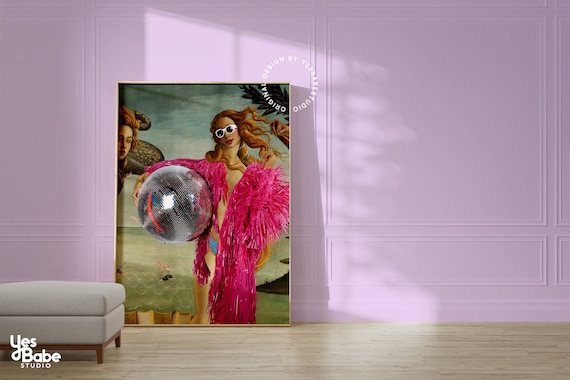In this vibrant room, the walls are painted a striking lavender hue with intricate crown detailing. The light wooden floor adds warmth to the setting. Dominating the left half of the image is a large, old-fashioned painting of two women, emphasizing one who is adorned with bold, modern accessories—a hot pink feather boa, white sunglasses, and a disco ball tucked under her arm, creating a vivid juxtaposition between classic and contemporary styles. The more prominent woman has wavy, light auburn hair, with a palm leaf subtly framing her head, seemingly at a beach scene with water in the background. A partial face of the second woman peeks from the left side of the painting. Resting against the wall near the painting is a cozy white ottoman. In the bottom left corner of the image, "Yes Babe Studio" is inscribed in elegant script, while a small circular watermark at the upper center reads "Original Design by Yes Babe Studio."